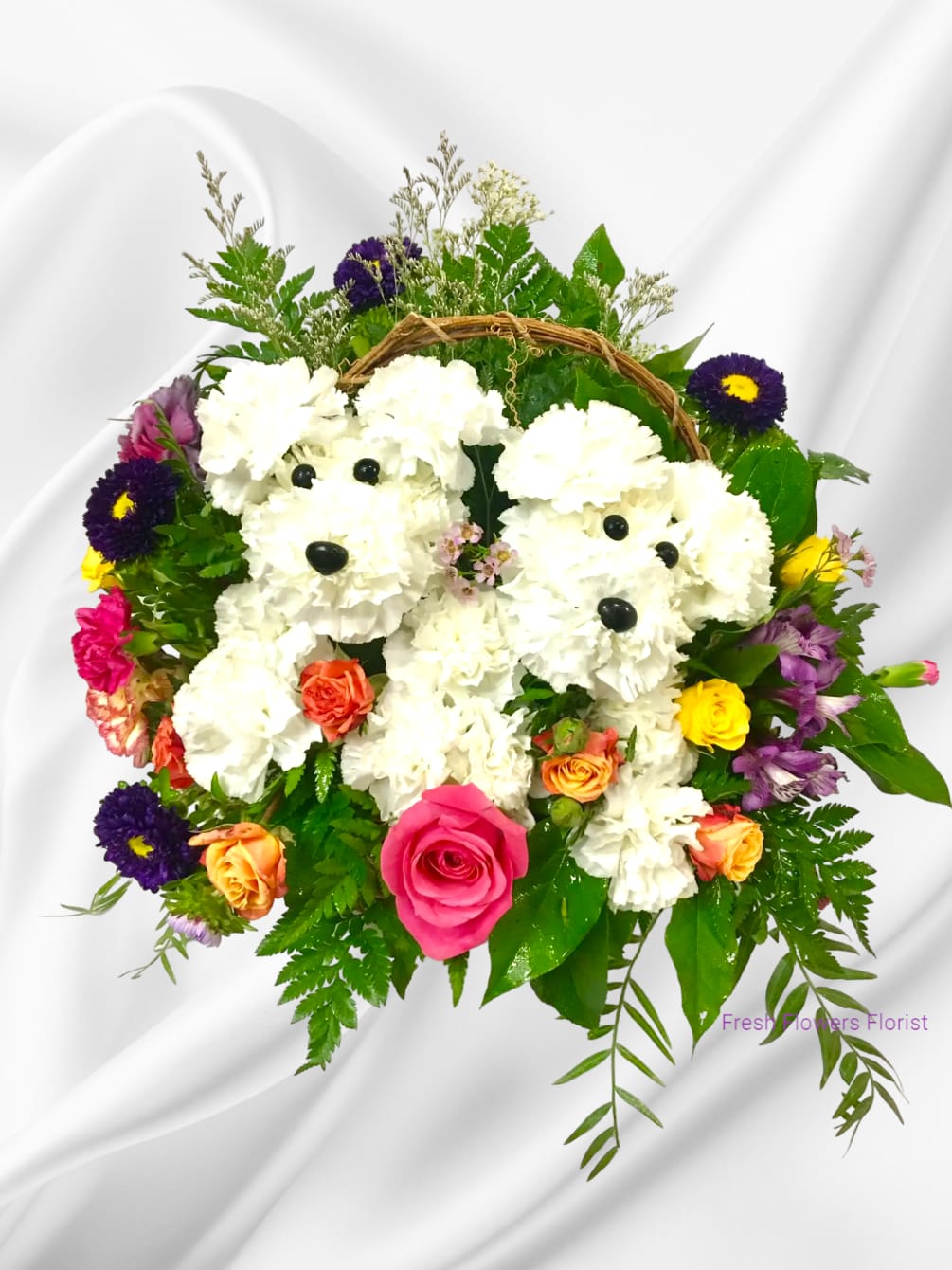This is a vibrant, color photograph of an intricate floral arrangement in a shallow basket, set against a white fabric background. The centerpiece of the bouquet is an artistic creation featuring two adorable puppy dogs made from white carnations. Each pup is intricately formed with rounded mounds of carnations for their faces, fluffy carnations for their ears, and elongated shapes at the front to represent their paws. Their faces are thoughtfully detailed with black buttons for eyes and noses, giving them a lifelike appearance. The puppies are surrounded by an abundance of green foliage, including ferns and large leaves, which provide a lush backdrop. Adding more bursts of color, the arrangement includes a red and pink rose at the bottom, smaller orange and yellow roses, and various blue, light purple, and purple flowers with yellow centers scattered throughout. To the left of the basket, "fresh flower florist" is written in a purple or lavender color, suggesting this image might be featured on a florist's website to showcase their artistic flower arrangements.